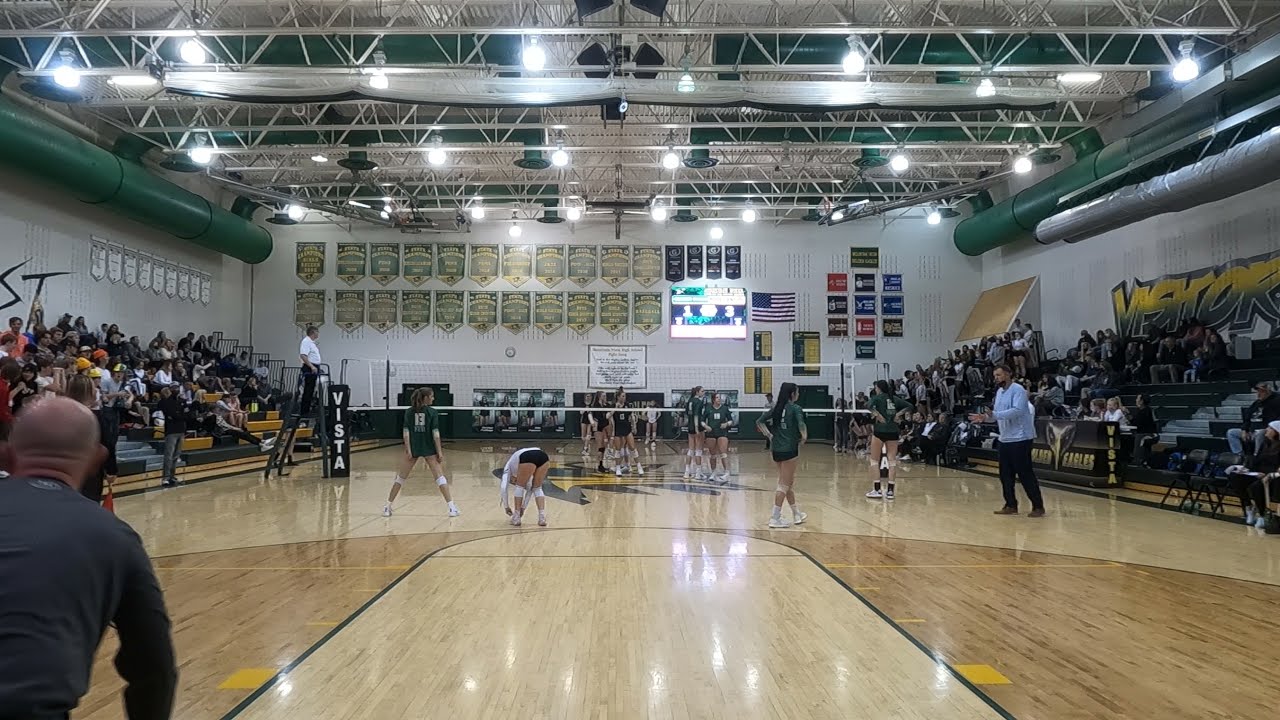This detailed, color photograph captures a high school gymnasium setting during an intense girls' volleyball game. The photograph is oriented in landscape, offering a clear view of the hardwood floor polished to a shiny finish, reflecting the bright white overhead lighting. At one end of the volleyball court, bleachers filled with spectators flank both sides, with the black bleachers on the right designated as the "visitor" section, indicated by green and yellow signage with black highlighting.

Players in green tops and black shorts compete energetically on the court. On the left side, a referee stands on a ladder-like stand, identifiable by a black vertical sign reading "VISTA" in white vertical lettering. The referee is dressed in black slacks and a short-sleeved white t-shirt, vigilantly overseeing the match. To the lower left corner, the back of a bald man, possibly a coach, is visible, wearing a long-sleeved gray t-shirt. Another man, also in black slacks but with a long-sleeved light-colored t-shirt, stands on the right side of the net, conversing with one of the players.

In the distant background above the visitor bleachers, an array of award banners and an American flag decorates the wall, adding to the school spirit captured in this lively indoor scene. The scoreboard indicates a score of 1-3 as the game progresses, encapsulating a moment of competitive fervor and community within the gym's tall, metal grid-work ceiling.